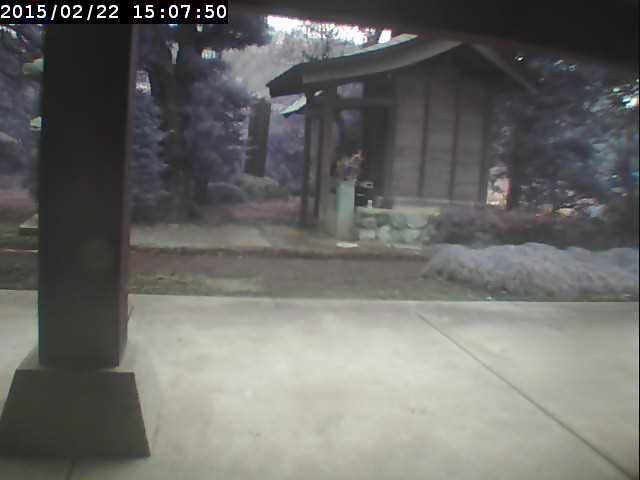Captured from a high vantage point, this image appears to be taken by a doorbell or security camera, possibly in a historical neighborhood in East Asia—either China or Japan. The focal point of the image is a wooden building adorned with an ornate, curved roof, characteristic of traditional East Asian architecture. The building is partially enclosed by a stone wall that borders the front premise. 

In the foreground, a large stone or cement pillar dominates the view, indicating the presence of a sidewalk along the street. The surroundings are lush, with numerous trees and bushes creating a verdant backdrop. The overall composition of the image is somewhat washed out, rendering colors indistinct. No text is visible within the frame, and the scene exudes a serene, timeless quality, reflective of its historical setting.